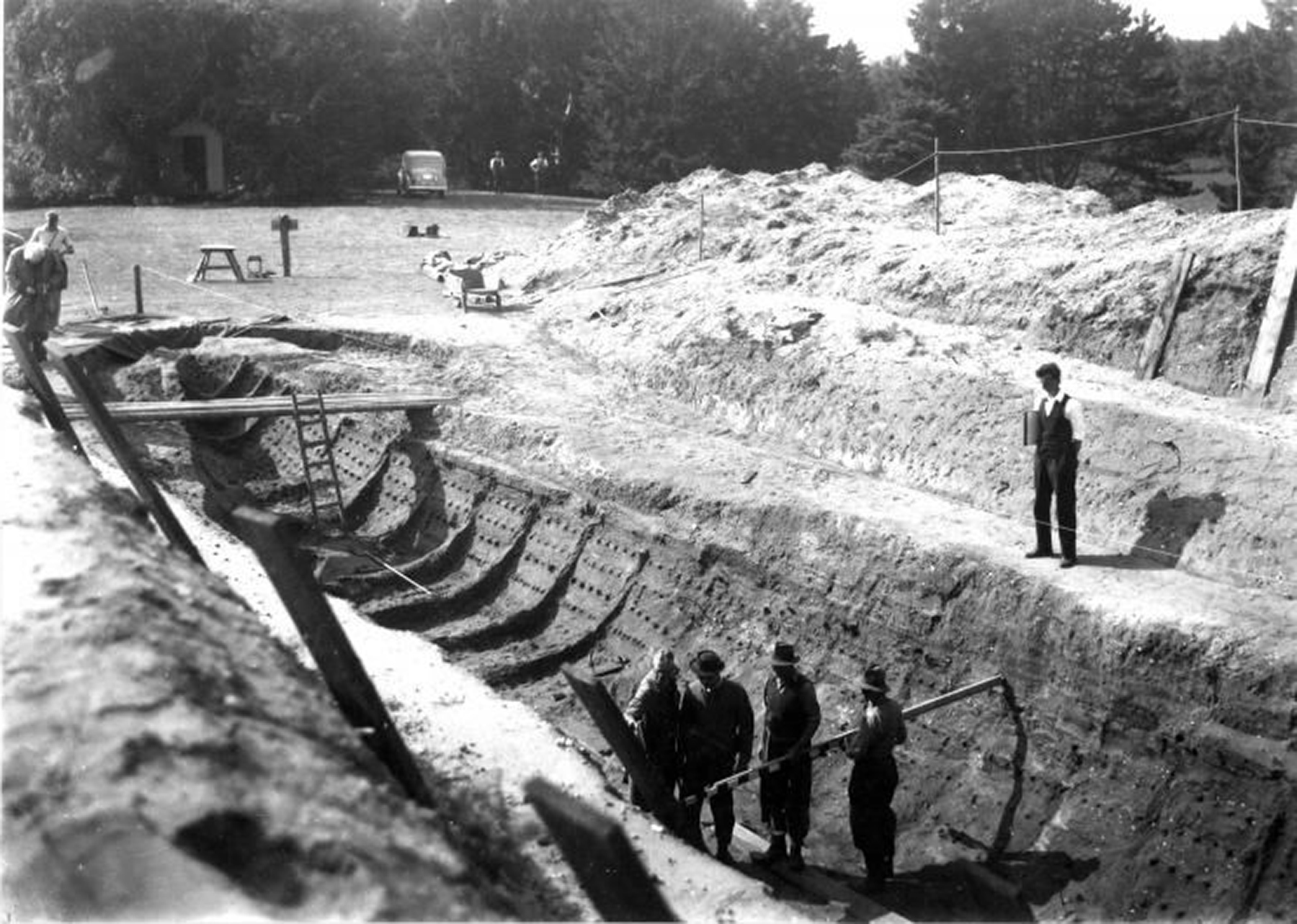In this black and white photograph, which is square and taken outdoors during the daytime, an archeological site is depicted with great detail. The upper portion of the image showcases a backdrop of trees with glimpses of the sky. Centrally and towards the upper section, two men stand beside a vehicle, appearing to be engaged in discussion. To the upper right, piles of excavated dirt cascade down multiple levels, creating a sense of depth and ongoing activity.

The central focus of the photograph is a pit where most of the excavation appears to be taking place. A man, dressed in a white collared shirt, dark vest, and long dark pants, stands at the edge of this pit, gazing down thoughtfully. Within the pit are four men, actively engaged in the excavation process. They are holding a pole, working together among several visible holes along the pit's walls. A wooden board and a ladder are strategically placed across the pit, indicating methods to navigate the site. The walls of the pit show features that resemble rivets, evoking the interior of a boat, adding an intriguing aspect to the scene. This richly detailed photograph captures the meticulous efforts of the men working at the archeological site, framed by the natural landscape and historical ambiance.